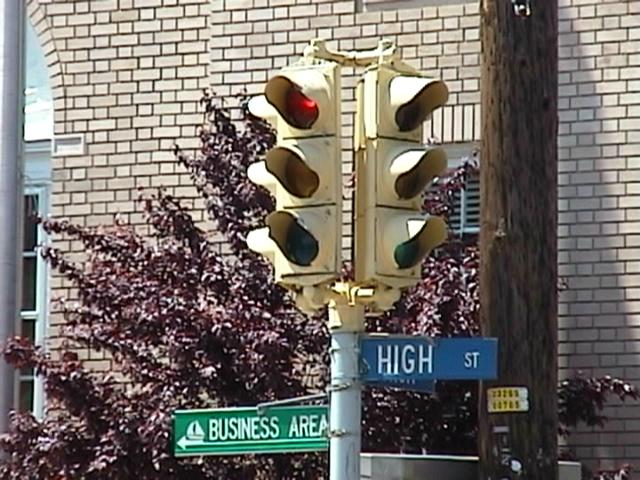This image captures a vibrant urban scene. Central to the photograph, taken outdoors, is a three-way yellow metal traffic light, clearly showing the illuminated green, yellow, and red lights. Behind this traffic light, a brick building stands prominently in the background. A wooden pole, likely serving as a power pole, is positioned at the front of the building, adorned with an unreadable yellow label. A striking purplish-red bush adds a splash of color to the scene. Below the traffic light, a blue and white road sign indicates "HIGH STREET," while a green sign with white lettering beneath it designates the "BUSINESS AREA," both written in capital letters. The overall photograph vividly captures the bustling character of this urban intersection.